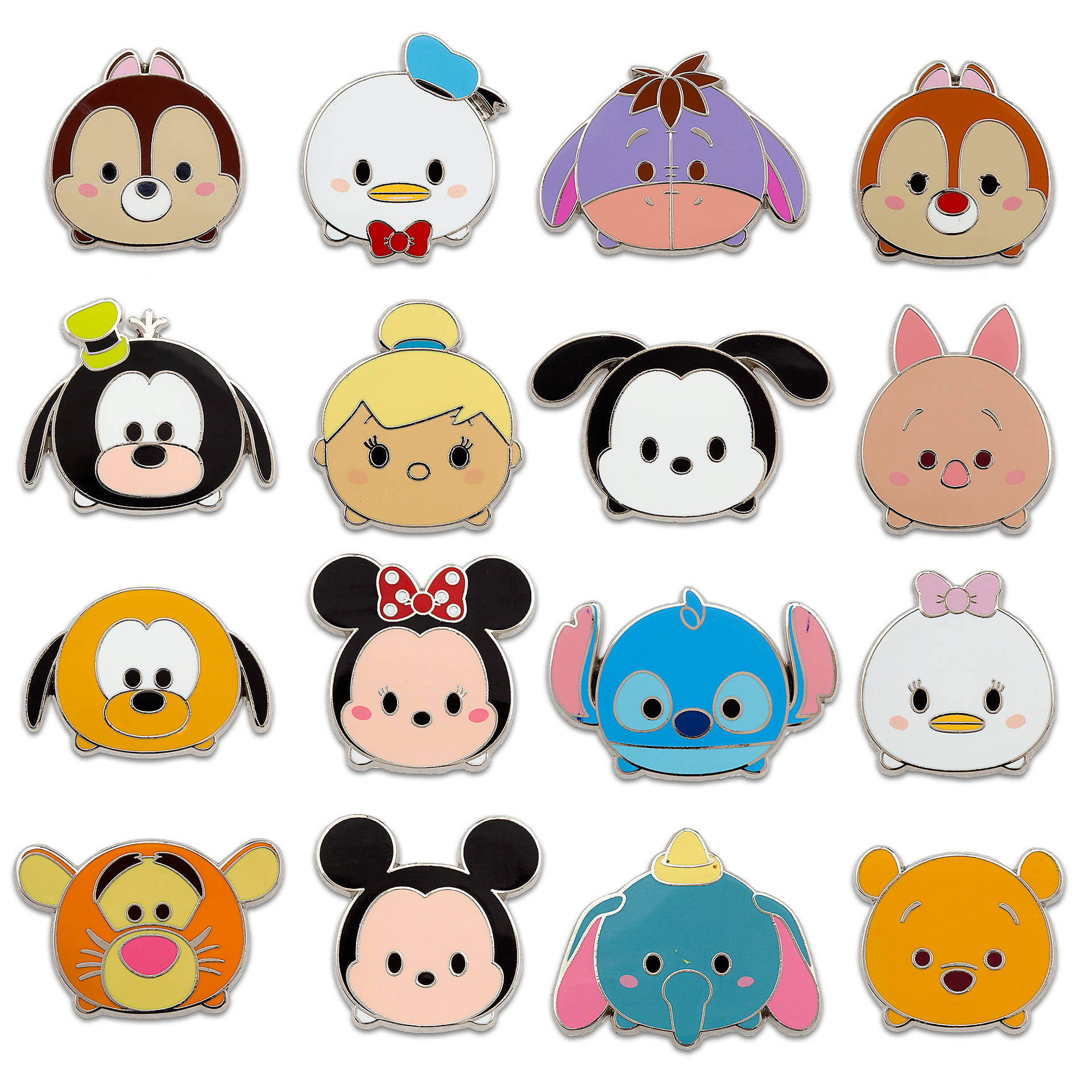This color photograph displays a collection of 16 colorful die-cast metal pins, arranged in four neatly organized rows. Each pin features the head of a beloved Disney character, portrayed in a cute, cartoon-like style with little tiny legs. These could serve as collectors' items or practical refrigerator magnets, given their flat design. Notable characters include a purple Eeyore, an orange Tigger, an orange Winnie the Pooh, a pink Piglet, a Mickey and Minnie Mouse, and a black and white Goofy with a yellow cap. In addition, there is a girl with blonde hair resembling Tinkerbell. The vibrant pins vary in hues of white, black, pink, yellow, blue, and purple, capturing the essence of Disney magic.